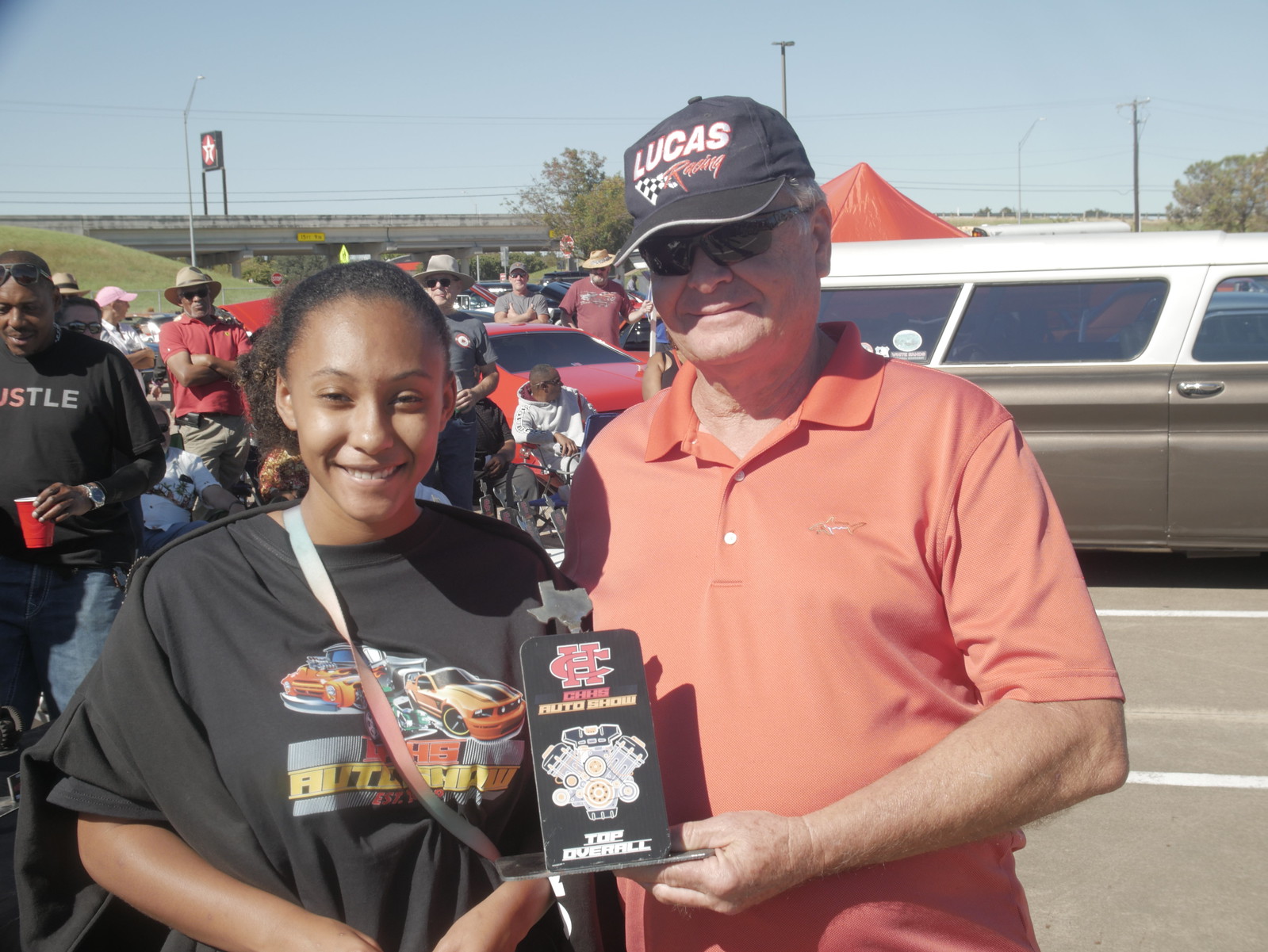In this vibrant outdoor image set at a bustling car show beneath a clear blue sky, an array of details captures the lively atmosphere. Dominating the foreground, a young black girl sports a graphic black T-shirt adorned with images of hot rods and sports cars. Standing beside her is an older, middle-aged white man with gray hair, clad in an orange polo shirt and a "Lucas Racing" baseball cap. He is also wearing sunglasses and proudly holding a black placard or trophy that reads "CH Cars Auto Show" with an engine block illustration and the title "Top Overall," topped with a small Texas-shaped metal piece.

In the background, a crowd of people engages in tailgating activities, sitting on foldable camping chairs and drinking from red Dixie cups, adding to the event's communal spirit. Among them, a man in a black T-shirt and blue jeans, also wearing glasses, can be seen smiling. A red car and a station wagon are parked nearby, with a red canopy tent and various signs, including a star-shaped highway sign and utility poles near a distant bridge, adding depth and context to the scene. The overall image vividly encapsulates a fun-filled, sunlit day at the fairground-like car show, teeming with people and classic automobiles.